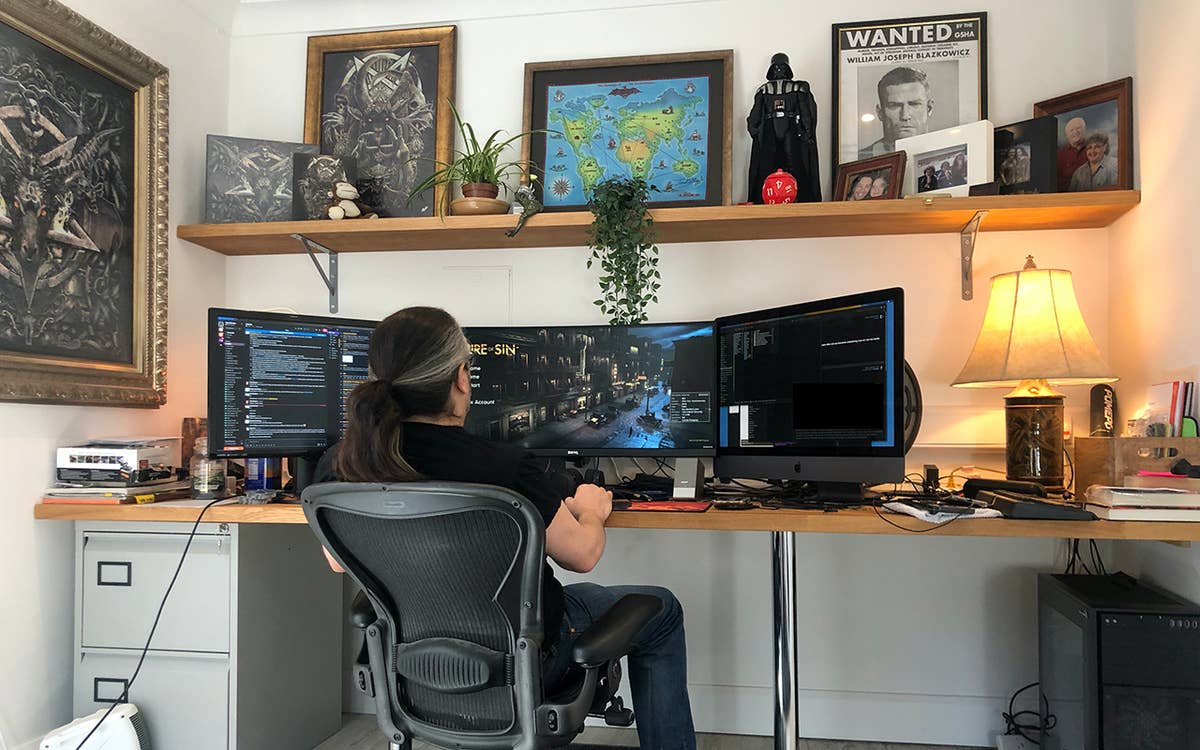In this detailed photograph, a man with long, dark hair tied in a ponytail, adorned with a few gray streaks, is seated in a computer chair at his cluttered wooden desk. The man, dressed in a black shirt and blue jeans, is working with a triple monitor setup. The central monitor is notably larger than the two flanking monitors, which display a mixture of tech codes and a computer game. The workspace is bathed in daylight, though a lamp is also on to his right. The desk is laden with numerous items, including additional keyboards, a joystick, a desktop computer with numerous trailing wires, and various books.

Against the white walls surrounding the area, the desk is supported on the left by beige filing cabinets. Above the desk, a floating shelf holds an eclectic assortment of personal items: a small potted plant, family photos, and framed art, as well as a distinctive art deco painting and a wanted poster for William Joseph Laskowitz. The shelf also features a Darth Vader statue. The floor beneath the desk, not fully visible, appears to be a dark-colored carpet. To the right, against the wall, a chrome pillar bolsters the desk setup, highlighting the practical yet packed nature of this personal workspace and gaming area.